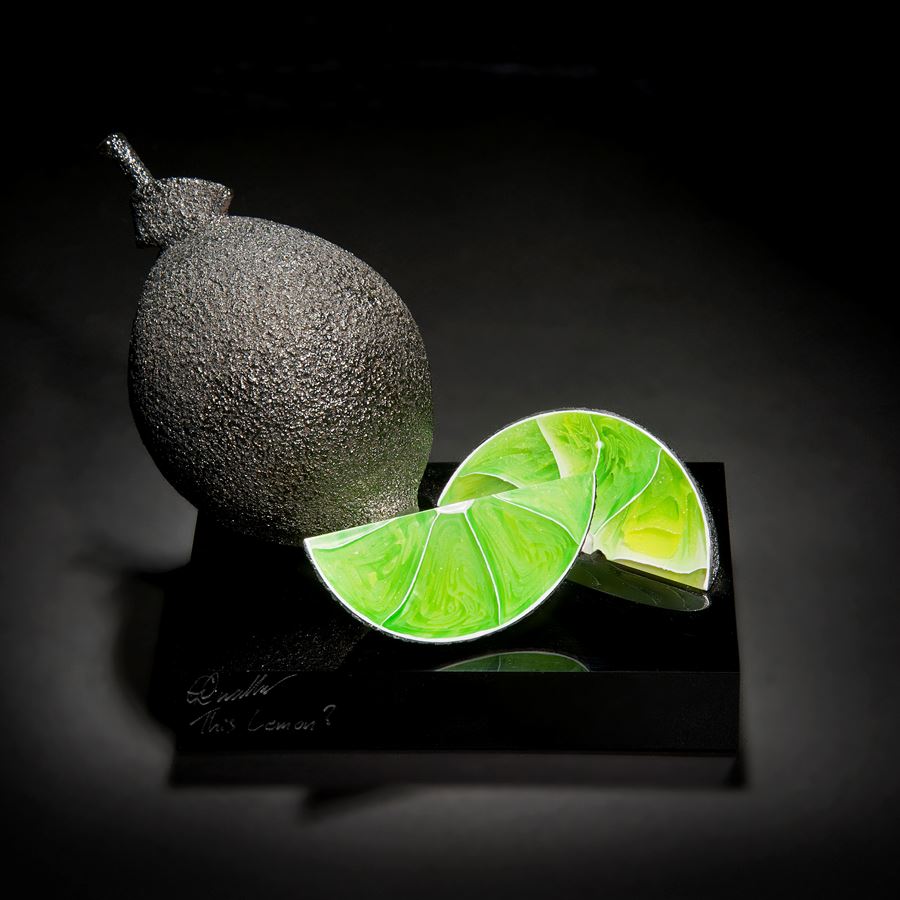The image is a detailed photograph of a well-lit sculpture featuring various lime elements. The centerpiece is a glossy black, book-thick square pedestal signed in white script on its lower left corner. On this base, there are two bright green lime wedges with distinct white pithy segment separators and a pithy area beneath the rind. The front lime wedge stands upright like a boat, while the slightly thicker wedge behind lays on its side, showcasing yellow marbling. Additionally, to the left side of the pedestal, there is a lime-shaped object sculpted to resemble a lime but made of cast iron with a mottled surface. It has a stem protruding from one end which doesn’t entirely align with traditional lime features, though the rest of the shape mirrors a lime. The background is a gradient of black and gray shadows, and the light source, emanating from the upper right just outside the frame, enhances the three-dimensional effect of the lime slices and the cast iron lime sculpture.